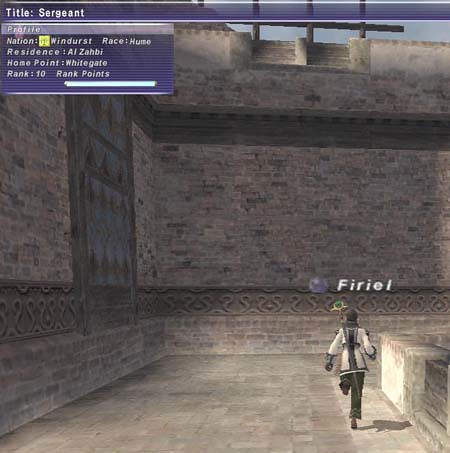This image showcases a digital drawing designed in a video game aesthetic. Dominating the top portion of the image is a blue information bar titled "Sergeant," beneath which lies a smaller blue box containing labels such as "Profile," "National," and an illegible country name, alongside an unreadable race, all seemingly fictional elements pertinent to the game.

The environment within the drawing exhibits medieval architectural influence, characterized by imposing flagstone walls that stand approximately six times the height of a human figure. These walls are composed of layered stone blocks and adorned with various decorative elements. Particularly noticeable is a metal design positioned about a quarter way down one wall, and a tapestry hanging on the left side, adding to the scene's historical ambiance. The base of the wall transitions into a decorative brick fence.

In the backdrop, castle-like turrets emerge, reinforcing the medieval fantasy setting. The lower third of the image features a paved road or path, extending across the scene's center. Alongside this path, on the far left, a character named "Fury L" is captured in motion. This figure, clothed in a white jacket and brown pants, appears to be running, adding a dynamic element to the tranquil medieval scene.